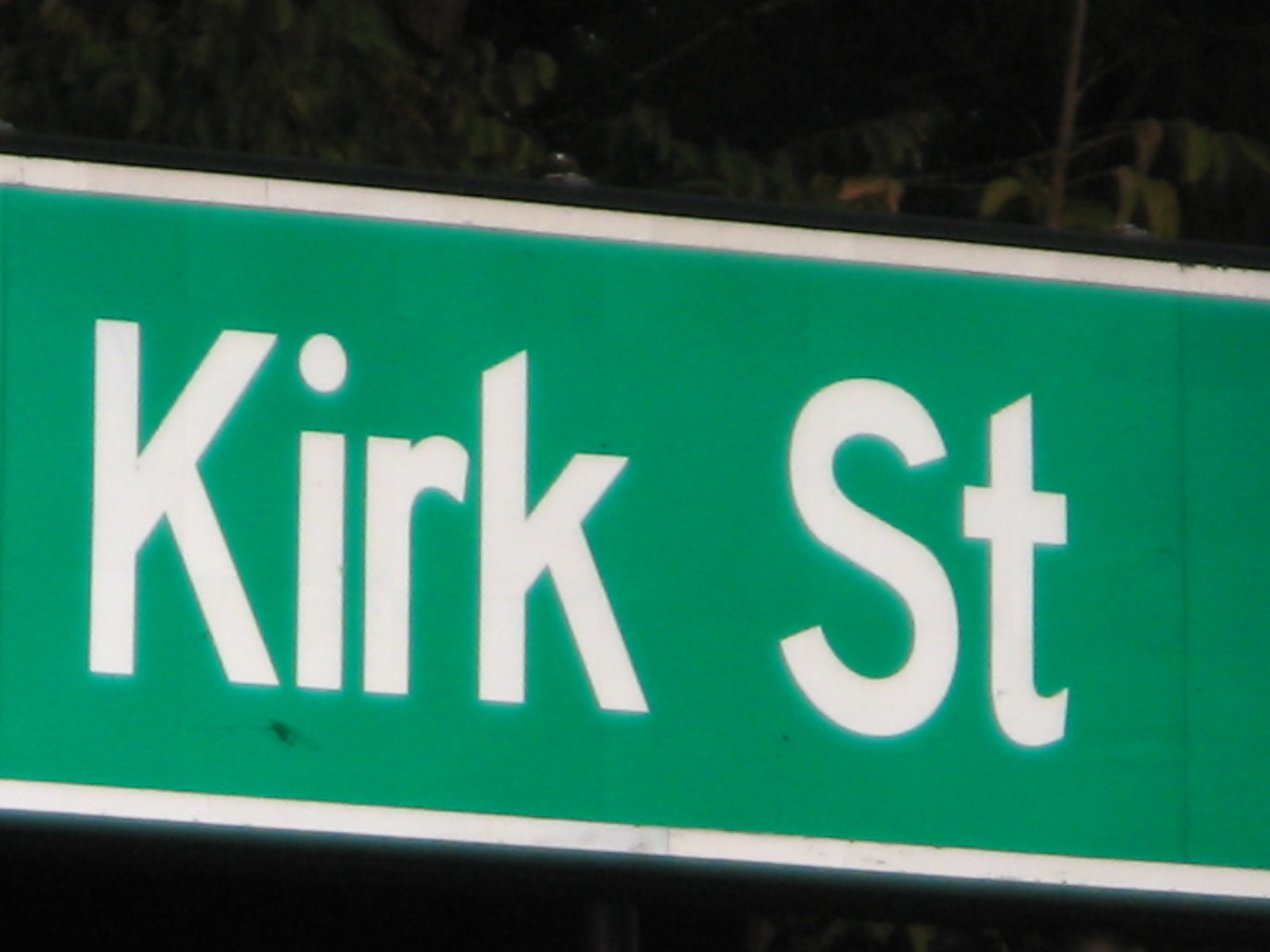This is an extreme close-up of a green street sign with white block letters reading "Kirk ST," featuring a white border along its edge. The sign displays slight weathering, particularly around the border, and a small black smudge beneath the letters "K" and "I." Due to the composition, not all of the sign is visible, revealing only the center and partial starts of the edges, especially on the right. The sign appears slightly tilted to the right. In the background, there are faint outlines of trees and leaves against a dark sky, indicating the photo was taken at night.